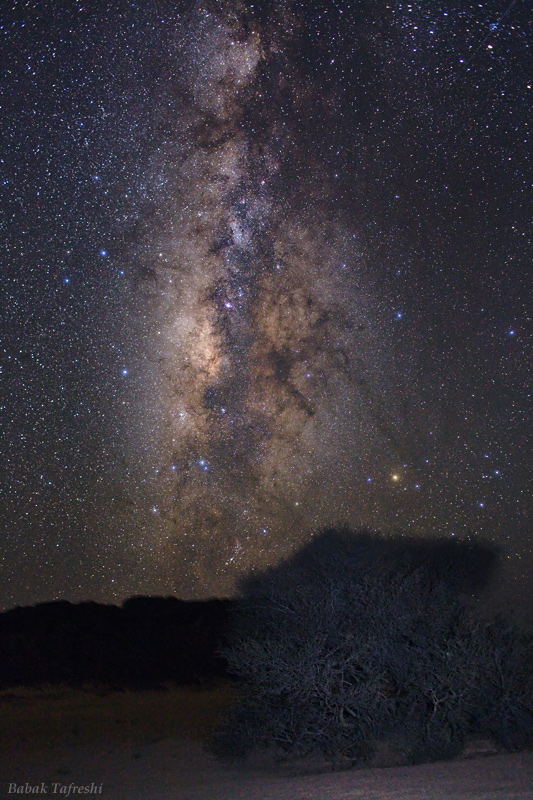The photograph captures the breathtaking view of the Milky Way galaxy in a vertical rectangular frame taken at night in a desert landscape. The dark black sky is adorned with numerous tiny white and light blue stars scattered across it. Running straight down the center, slightly angled towards the bottom, is the Milky Way—a striking blend of dark and light purple hues, surrounded by a haze of light yellow, gray, and even some light orange and white shades. The detailed, vibrant nebula-like cloud adds a stunning focal point to the image. At the base of the picture, the ground appears a dark gray due to the night setting, with the silhouette of what seems to be a dark gray shrub and a dim ridge or possibly a line of trees in the background. The lower left corner displays a watermark crediting the photographer, Bob Bob To Freshie, enhancing the authenticity of this celestial masterpiece.